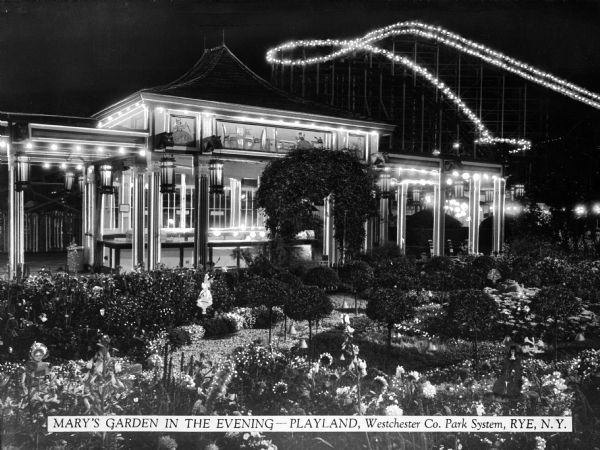The black-and-white image titled "Mary's Garden in the Evening, Playland, Westchester County Park System, Rye, New York," depicts a nighttime scene at a fair or theme park. In the foreground, we see a well-maintained garden with various plants and flowers, subtly illuminated, creating an inviting atmosphere. Standing prominently within the garden is a large, boxy structure, reminiscent of an old house, adorned with strings of white holiday lights outlining its windows, columns, and supporting beams. To either side of the building are spacious, flat-roofed porches supported by columns, adding to the architectural charm. In the distance, looming behind this illuminated building, is the distinct outline of a roller coaster, also lined with lights, further contributing to the festive ambiance of the scene.